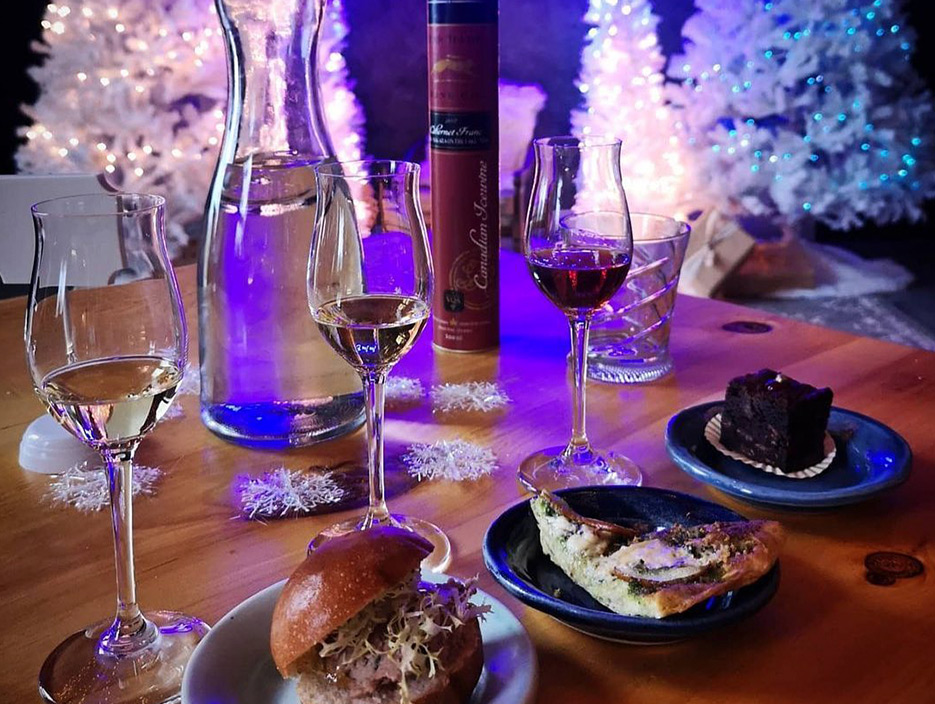On a beautifully set wooden table decorated for an elegant meal, three fluted wine glasses are positioned—two containing white wine and one filled with red wine. Each glass is paired with a different plate, arranged from left to right: A white plate holds a burger or sandwich made with a pretzel bun and topped with lettuce. A blue plate in the center presents a slice of quiche or frittata, while another blue plate at the far right features a rich, chocolate brownie, resting on a coffee filter-like paper. Adding to the ambiance, a bottle of wine and a carafe of water sit prominently on the table. In the background, white Christmas trees embellished with sparkling lights cast a festive glow against a dark-colored wall, enhancing the celebratory atmosphere. A delicate white snowflake ornament also embellishes the table, enhancing the overall holiday charm.